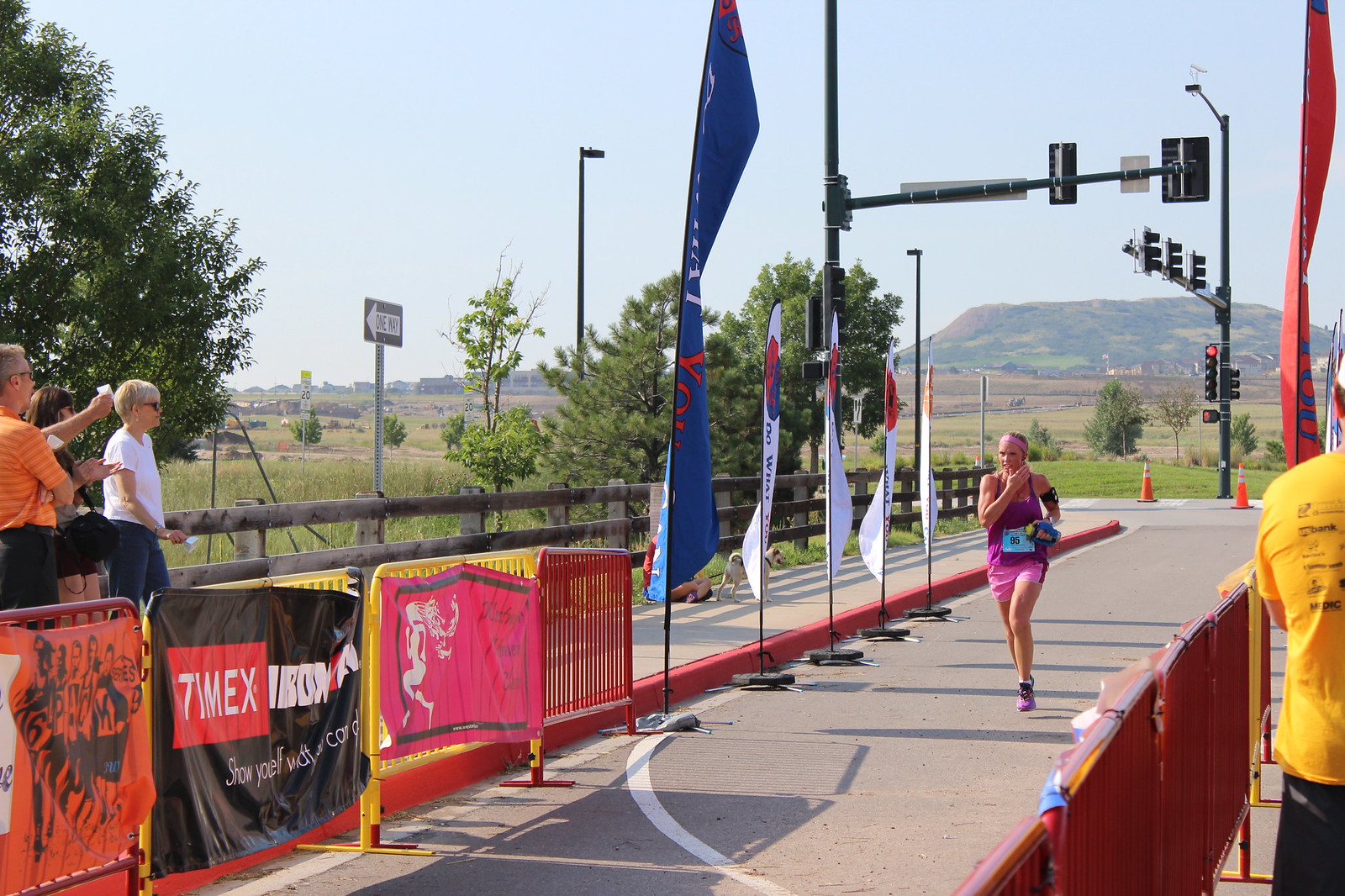In the image, taken outside on a sunny day under a clear blue sky, a woman is captured running towards the camera in what appears to be a road race or marathon. She is wearing a purple tank top and purple shorts with a pinkish hue. The racecourse, which looks like a wide sidewalk or narrow road, is lined with red fencing and various banners, including a red banner on the right and a blue banner on the left. The lane is further bordered by metal fencing and partitions, guiding the runners towards the finish line.

To the left of the image, there is a tree in the upper left corner, partially visible. Adjacent to the tree is a one-way traffic sign nestled within wooden fencing. On the right side of the image, in the background, there is a lush mountain or large hill blanketed with greenery. An intersection with traffic lights is also visible in the distance, with one light showing red.

A few spectators are gathered along the left side of the course, cheering on the runners. In the middle of the image, banners reading "Timex" are prominently displayed. The scene is bustling with activity and supportive onlookers, highlighting the spirited atmosphere of the race.